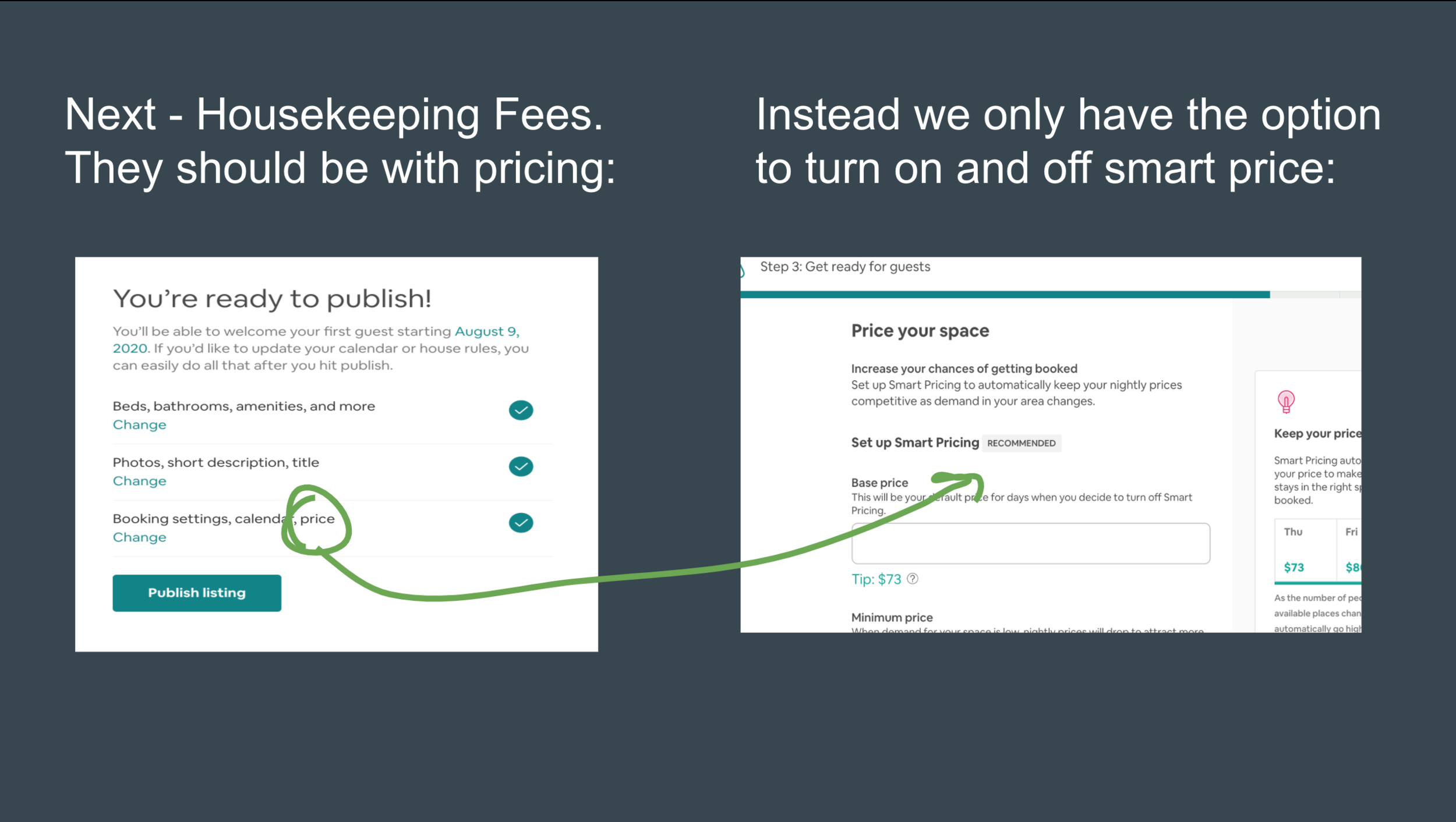In this tutorial-style image, two screenshots are placed against a navy gray background to provide guidance for users listing their properties on a platform resembling Airbnb. The header text, "Next, housekeeping fees should be with pricing. Instead, we only have the option to turn on and off smart price," indicates a key area of concern regarding pricing settings. 

The first screenshot highlights the prompt, "You're ready to publish. You'll be able to welcome your first guest starting August 9th, 2020. If you'd like to update your calendar or house rules, you can easily do that after you hit publish." This section includes elements such as beds, baths, amenities, photos, short descriptions, titles, booking settings, calendar, and price, with the word "price" circled in green. There's a clear instructional angle, marked by an arrow leading to the second image to emphasize continuity.

In the second screenshot, the text "Price your space, increase your chances of getting booked. To set up smart pricing automatically, keep your nightly prices competitive as demand in your area changes," appears, promoting the use of smart pricing. However, the user's frustration is evident as the tutorial underscores that the only available option is smart pricing, with no alternative to manually set prices. This detailed depiction helps clarify the steps and options—or lack thereof—currently available to property listers.